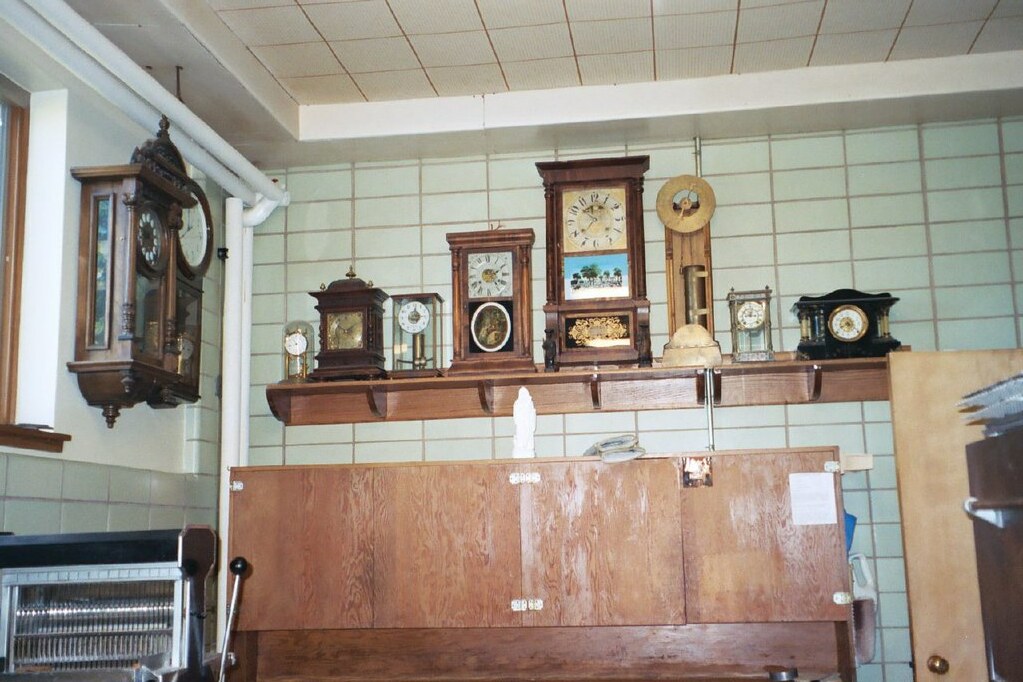The photograph depicts an interior room showcasing an eclectic collection of clocks. Dominating the scene is a brownish-red wooden shelf affixed to a greenish tiled wall with tan grout. The shelf holds a diverse assortment of approximately eight clocks, each unique in shape and size, ranging from an ornate square wooden clock and a black rectangular clock to round glass-encased timepieces. Below the shelf, a piece of plywood is visible, creating a two-tiered shelving effect with additional brownish-red wood at the bottom. The left side features two antique grandmother clocks mounted on a partial white wall partition. The upper part of the image reveals a white ceiling with tiles, detailed with light brown accents between them. White pipes traverse the ceiling, contributing to the room's industrial feel. On the far right, an open brown door with a bronze handle adds a touch of warmth, while a greyish cabinet sits unobtrusively at the bottom right. The scene is subtly framed by a white L-shaped molding running along the ceiling's edge, enhancing the room’s quaint yet functional atmosphere.